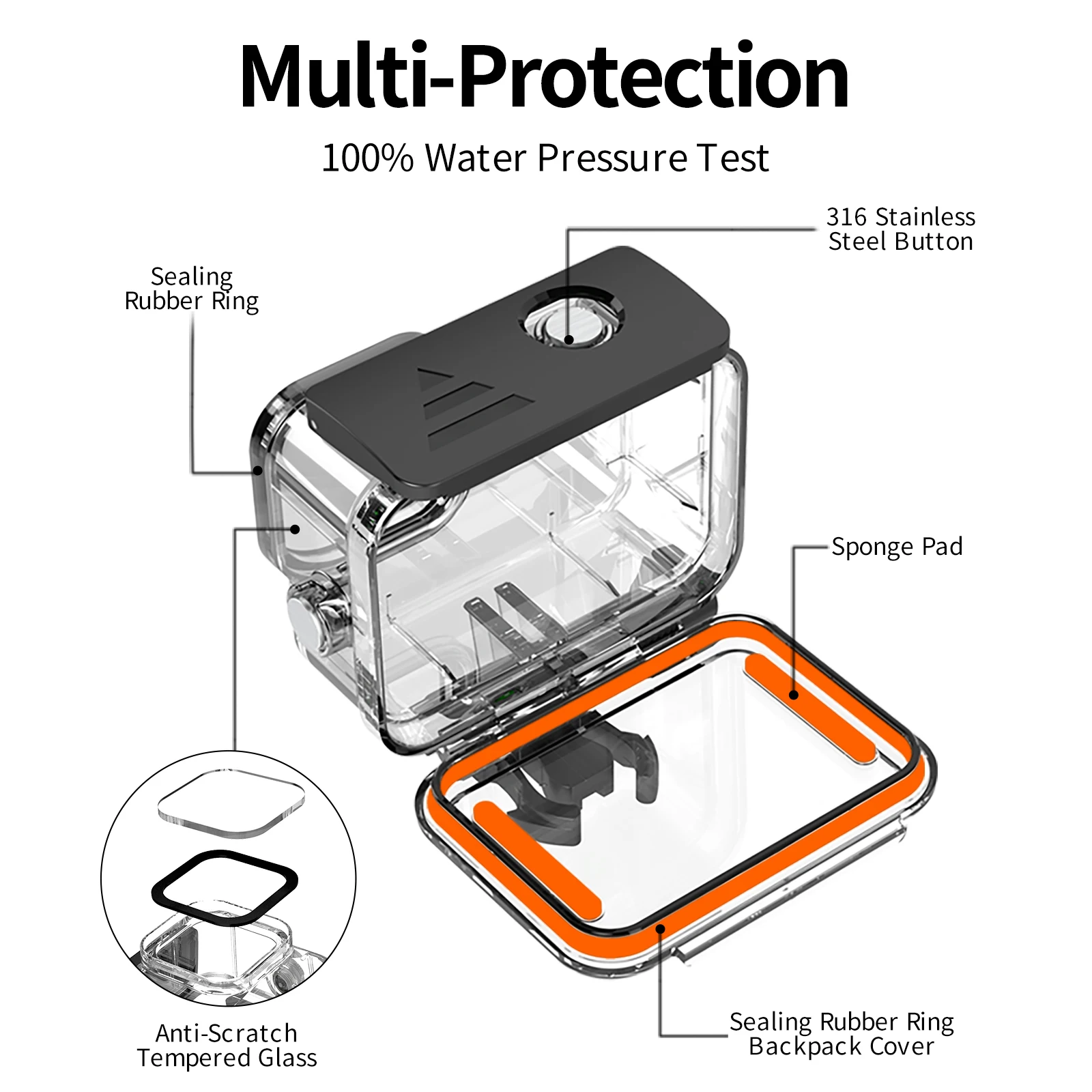The image showcases a transparent, clear enclosure designed for a GoPro camera, set against a white background. At the top of the image, it prominently displays the phrases "multi-protection" and "100% water pressure test" in bold black letters. The enclosure appears to be constructed from anti-scratch tempered glass with various labeled components. It features a black lid with a hole for the 316 stainless steel button, a sealing rubber ring for enhanced waterproofing, and a sponge pad located within the lid to secure the camera. Additionally, there is a sealing rubber ring back pad cover around the closing door. The overall design emphasizes durability and protection, ensuring the GoPro's safety from water and physical damage. The enclosure includes black and orange seals to provide extra security against leaks and impacts.